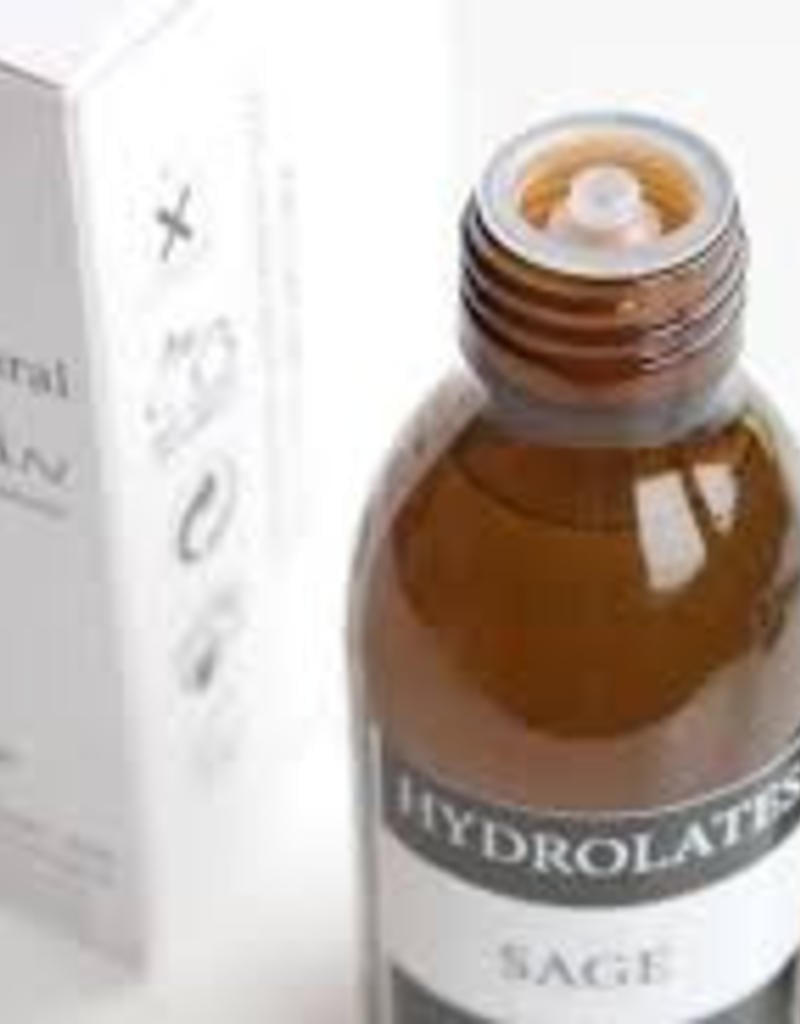The image depicts a slightly blurry product page featuring a brown glass bottle of aromatherapy oil prominently displayed against a light white background. The bottle, which is fitted with a dropper-style dispenser, is filled with a liquid scent and labeled in a distinctive black-and-white format. The label clearly reads "HYDROLATES" in white letters on the black portion, with "SAGE" in black letters on the white portion below, indicating that it is indeed sage-scented oil. To the left of the bottle, about a third of a white box is visible, featuring several logos and symbols related to the product. This box, which holds directions for use, complements the primary focus of the image—the brown bottle of sage aromatherapy liquid designed for use in diffusers to enhance room fragrance. Together, the bottle and the partially visible box occupy around eighty percent of the image, highlighting the product in a website advertisement setting.